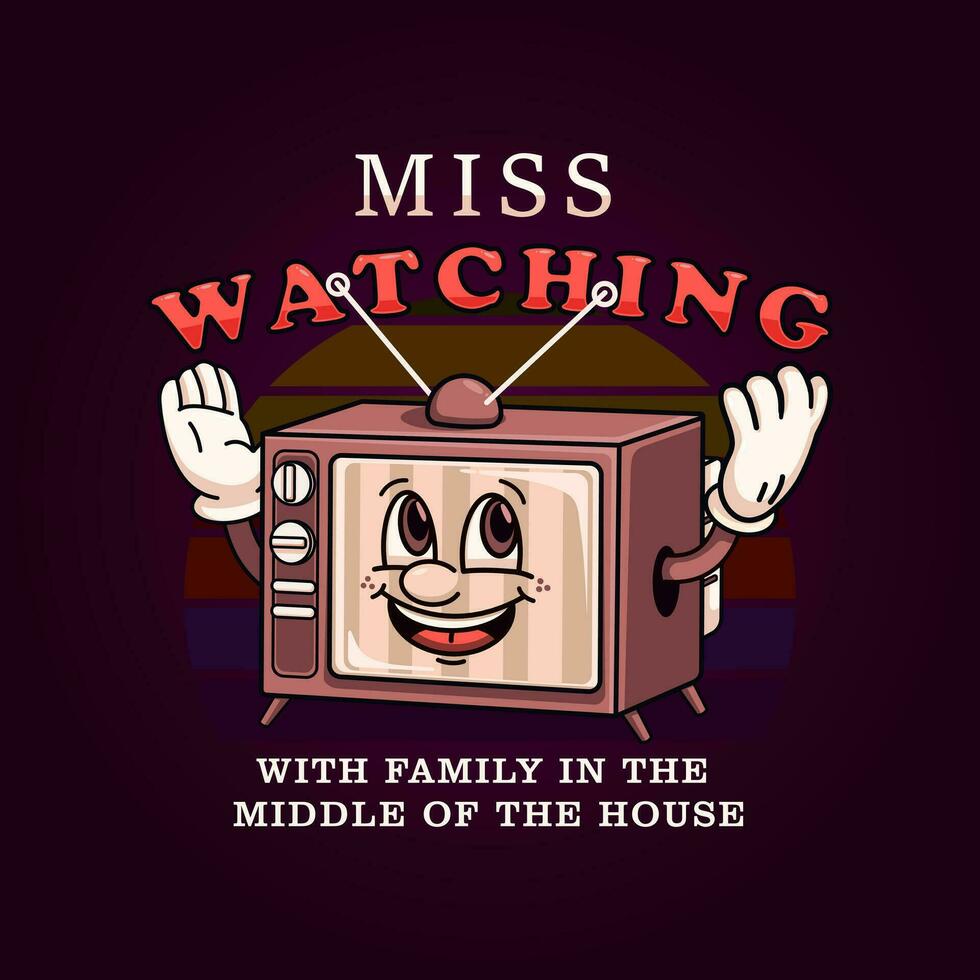The image is a detailed cartoon graphic featuring an old-fashioned tube television with a cheerful face. The background transitions from a black at the top to a dark blue towards the middle and bottom, giving a gradient effect. The text at the upper part of the image is in a mixture of white and pinkish hues for the word "MISS," and bold red letters spell out "WATCHING." Behind the TV, there is a circular pattern with striped rainbow colors that fade from green to navy blue, further blending into the background.

The TV itself is designed with vintage elements, including antennas on top, a channel tuner, a UHF tuner, and a side panel with multiple buttons. The TV's screen features a happy face with two eyes, a nose, dimples, and a smiling mouth, giving it an animated, friendly appearance. The TV also has arms extending from its sides, each adorned with white gloves reminiscent of Mickey Mouse’s gloves, raised up as if waving or celebrating. 

Below the TV, the text "WITH FAMILY IN THE MIDDLE OF THE HOUSE" is written in white letters. The entire scene seems to evoke a nostalgic sentiment, possibly encouraging or reflecting on the joy of watching TV with family at home.